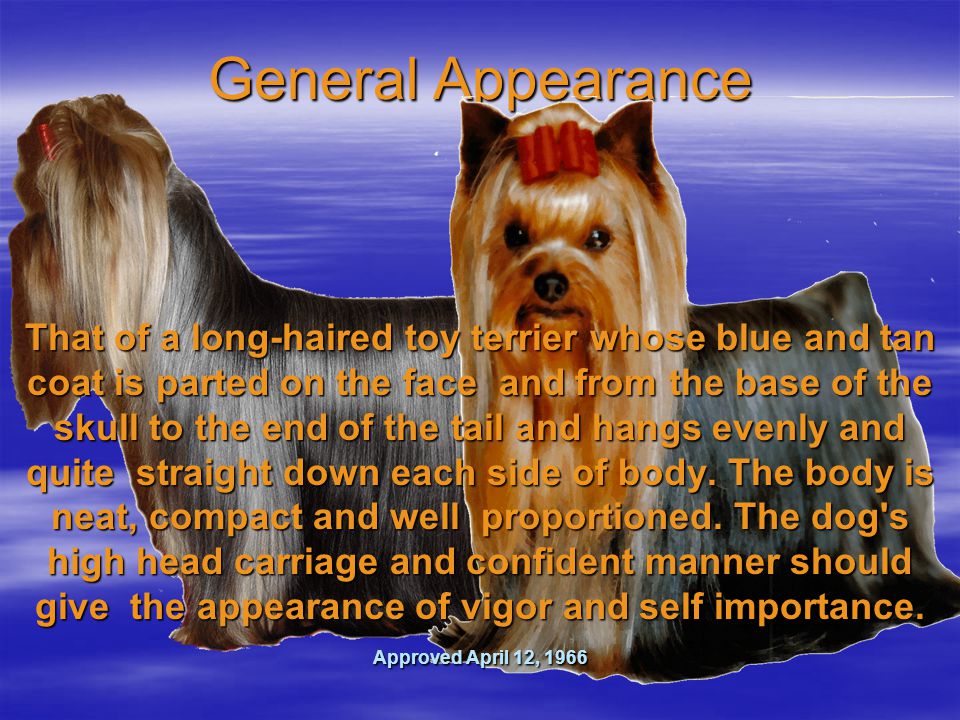The image appears to be a PowerPoint slide with an indigo blue background subtly streaked with white. At the top center, in bold orange letters with a black shadow, the title "General Appearance" is prominently displayed. Beneath this title are two photographs of a small, neatly groomed toy terrier. The left photo shows the dog in full profile, facing left, while the right photo presents the dog angled towards the viewer, adorned with a red bow in its hair. The dog's coat displays a mix of light brown, dark brown, black, and white colors. Superimposed over the images is detailed text in orange lettering, reading: "That of a long-haired toy terrier whose blue and tan coat is parted on the face and from the base of the skull to the end of the tail, and hangs evenly and quite straight down each side of the body. The body is neat, compact, and well-proportioned. The dog's high head carriage and confident manner should give the appearance of vigor and self-importance." In small, light blue text at the bottom, it notes, "Approved April 12, 1966."